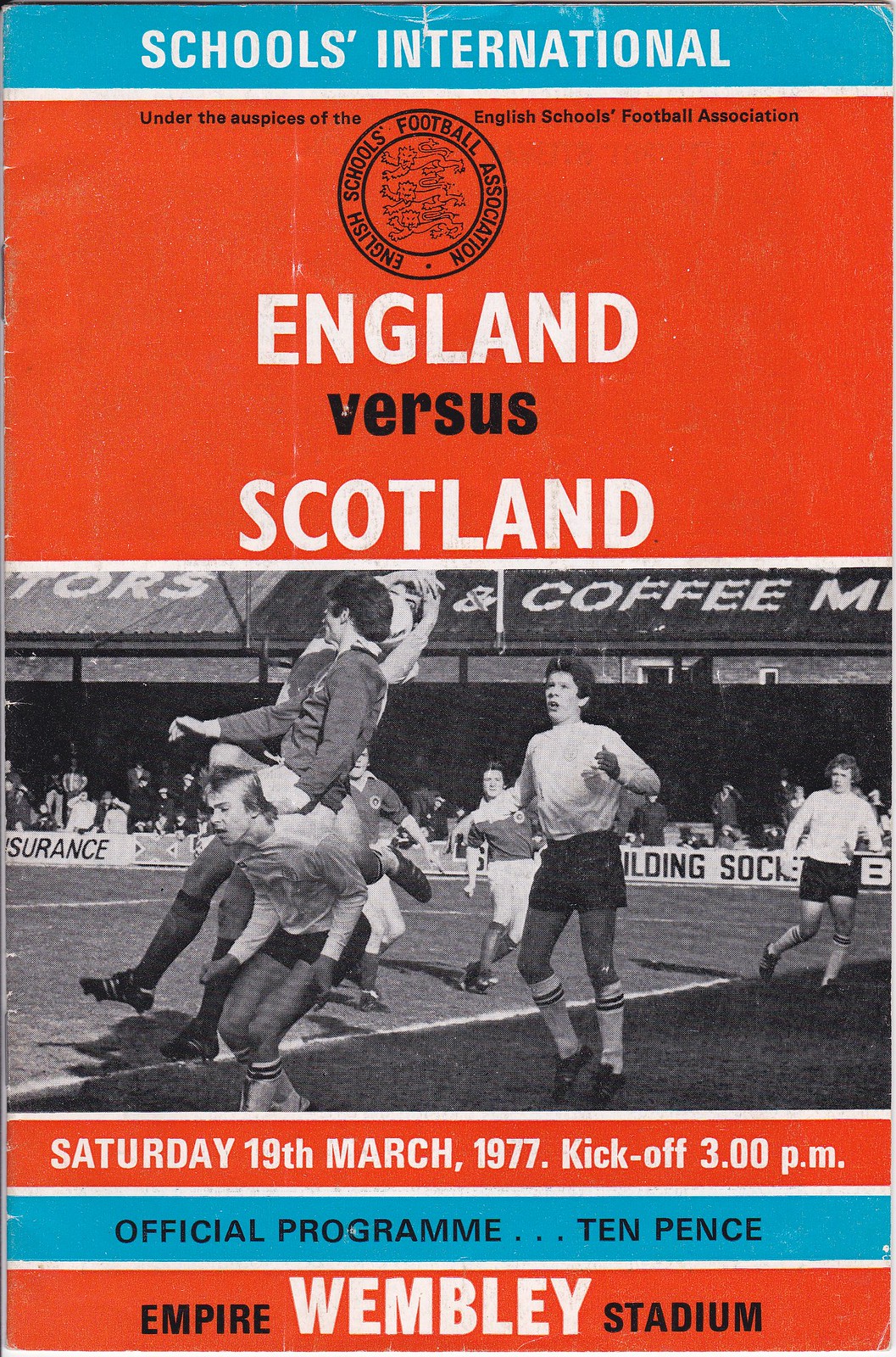This image is the cover of an official soccer program from the 1970s, dominantly featuring the colors blue, red, and white, with some black elements. At the top, a blue horizontal strip with white text reads "Schools International." Below this, a wider red horizontal strip displays the English Schools Football Association logo and announces "England vs Scotland" in large white letters, with the word "versus" in contrasting black text. Centered under the red strip is a black-and-white action photograph of players engaged in a soccer match. Beneath the photograph, another red horizontal strip in white text details "Saturday, 19th March, 1977, kick-off 3.00 pm." Following this, a blue horizontal strip with black writing declares the price, "Official Programme...10p." Finally, at the bottom, a red horizontal strip with the words "Empire Wembley Stadium" is featured, with "Wembley" prominently displayed in larger white lettering.